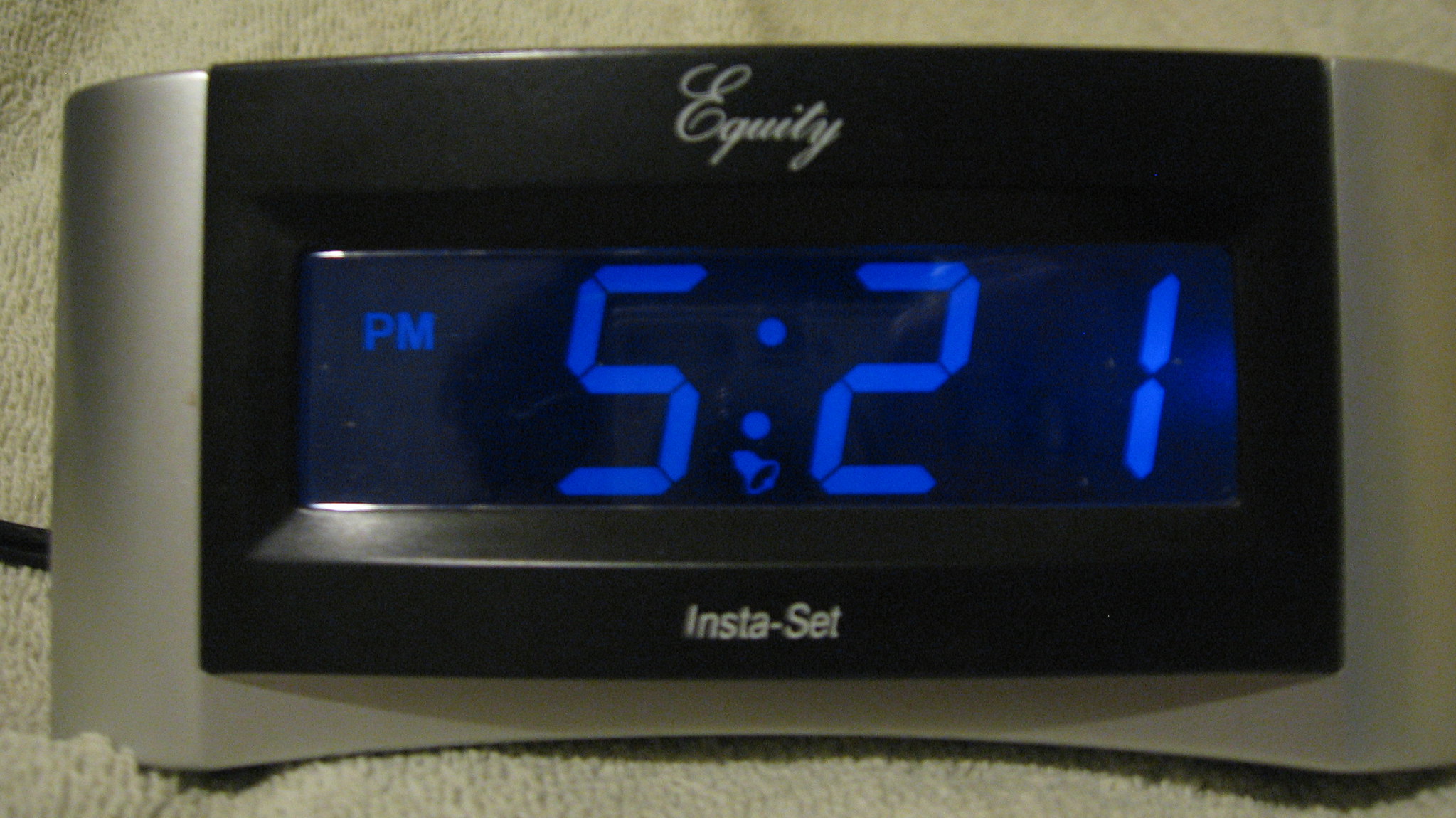This image features a bedside clock prominently displayed on a soft, cream-colored blanket with a hint of tan. The blanket appears to be fuzzy, suggesting a cozy texture. The clock itself is predominantly black with a wide, robust silver border that gives it a modern, sleek appearance. The time shown on the clock is 5:21 PM, with the numbers brightly illuminated in an eye-catching blue. The brand name "Equity" is elegantly written in white cursive at the top of the clock face, while the term "Instaset" is printed at the bottom, indicating a possible feature of the clock. This detailed snapshot captures the essence of a stylish yet functional timepiece in a comfortable setting.